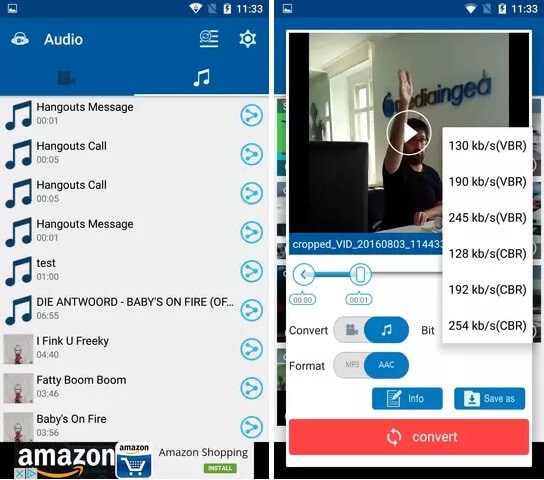The image comprises two screenshots captured from a mobile device, possibly a smartphone or tablet, as indicated by the presence of the time, battery, Wi-Fi, and service indicators at the top of the screen. Both screenshots display the time as 11:33 AM.

On the left screen, the interface features a predominantly blue and light gray color scheme, with black text. The screen appears to be an audio management interface, as suggested by the highlighted music note icon and various audio-related settings. Icons and settings, including a settings wheel and a music note, are visible at the top. Below these icons, a list of audio items is shown, including "Hangouts Message," "Hangouts Call," "Hangouts Call," "Hangouts Message," "Test," and three songs from Die Antwoord: "I Think You Freaky," "Fatty Boom Boom," and "Baby's on Fire." At the bottom of this screen is an advertisement for Amazon Shopping.

The right screen depicts a different interface, featuring a preview image of a man with his hand raised and a play button overlaying the image, indicating it is a video or multimedia file. Below this preview are options for converting the file, including a prominent red "Convert" button. Next to this button is a dropdown displaying various bitrate options: 130 KB, 190 KB, and 245 KB, suggesting different quality levels for conversion. The highlighted bitrate button indicates the user is focusing on selecting the desired conversion quality.